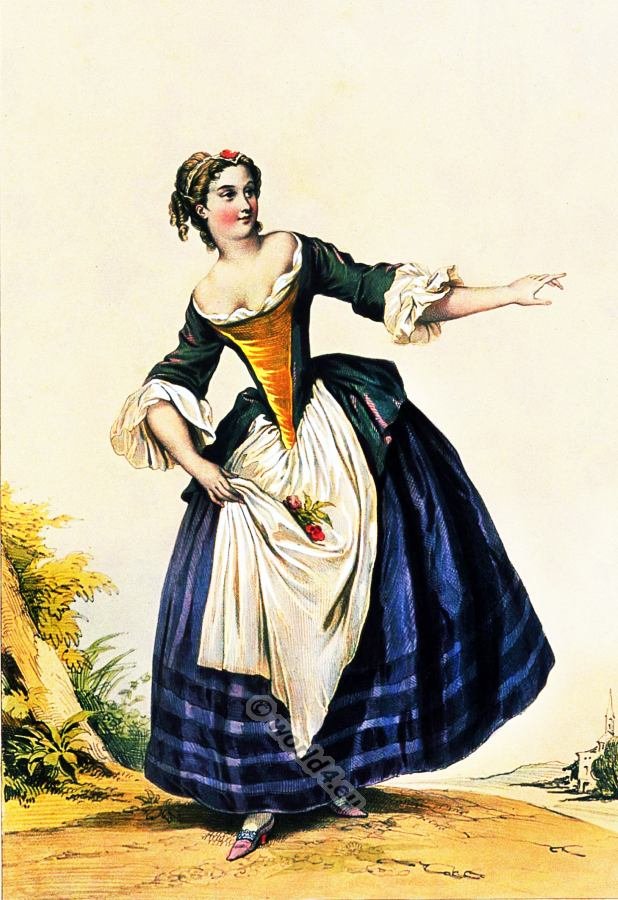This detailed illustration or painting depicts a fair young maiden in an elaborate outdoor scene. She is adorned in a striking, full-skirted, royal blue dress reminiscent of a ballroom gown, flaring dramatically at the bottom. The dress features darker blue stripes and has a light blue ribbon circling the hem, which sweeps down to her ankles. Over her dress, she wears a white apron, seemingly adorned with berries, gathered and tied at her narrow waist, which is further accentuated by a built-in corset or a similar form-fitted structure, making her waist appear extremely thin. The top section of her dress is green, off the shoulder, and embellished with a gold fabric insert that extends from her bust to a point at her waist. Her sleeves, falling just past her elbows, end in white ruffles, leaving her forearms bare. Her hair is elegantly styled up, with a few curly ringlets escaping, and is accessorized with a headband and a red and white headpiece. The maiden's skin is rosy-cheeked, possibly due to makeup, and she glances to the right, pointing in the same direction with her left hand. She is poised on a dirt path, surrounded by various elements of nature, including a tree stump, some rocks, greenery, and a hint of a church spire visible in the lower right background. Her ensemble is completed with pointed pink shoes featuring small heels.